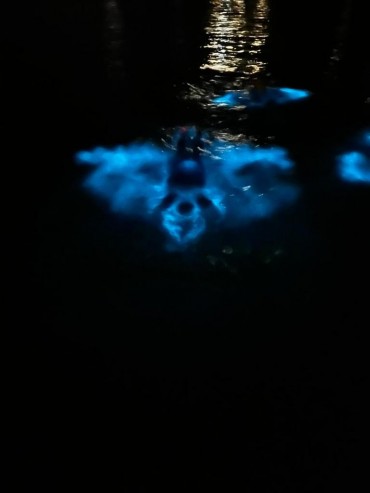In this dark and ominous image, the scene is predominantly black, creating a mysterious and eerie atmosphere. In the upper right-hand side of the photo, a brown object can be spotted, though it's unclear whether it is an actual item or a reflection, adding to the photo's ambiguity. A light source in the background casts minimal illumination, revealing ripples on the surface of what appears to be water. Floating in the dark water, there are several vibrant blue shapes. One shape resembles a small, bright blue moth or butterfly with detailed wings and a body, while another is an abstract, elongated form with vibrant blue ends. The most striking detail is the presence of a frightening figure formed in the reflections—an ominous, skeletal dog-like face seemingly staring out, surrounded by a blue haze. These elements combine to create a highly unsettling and mysterious visual.